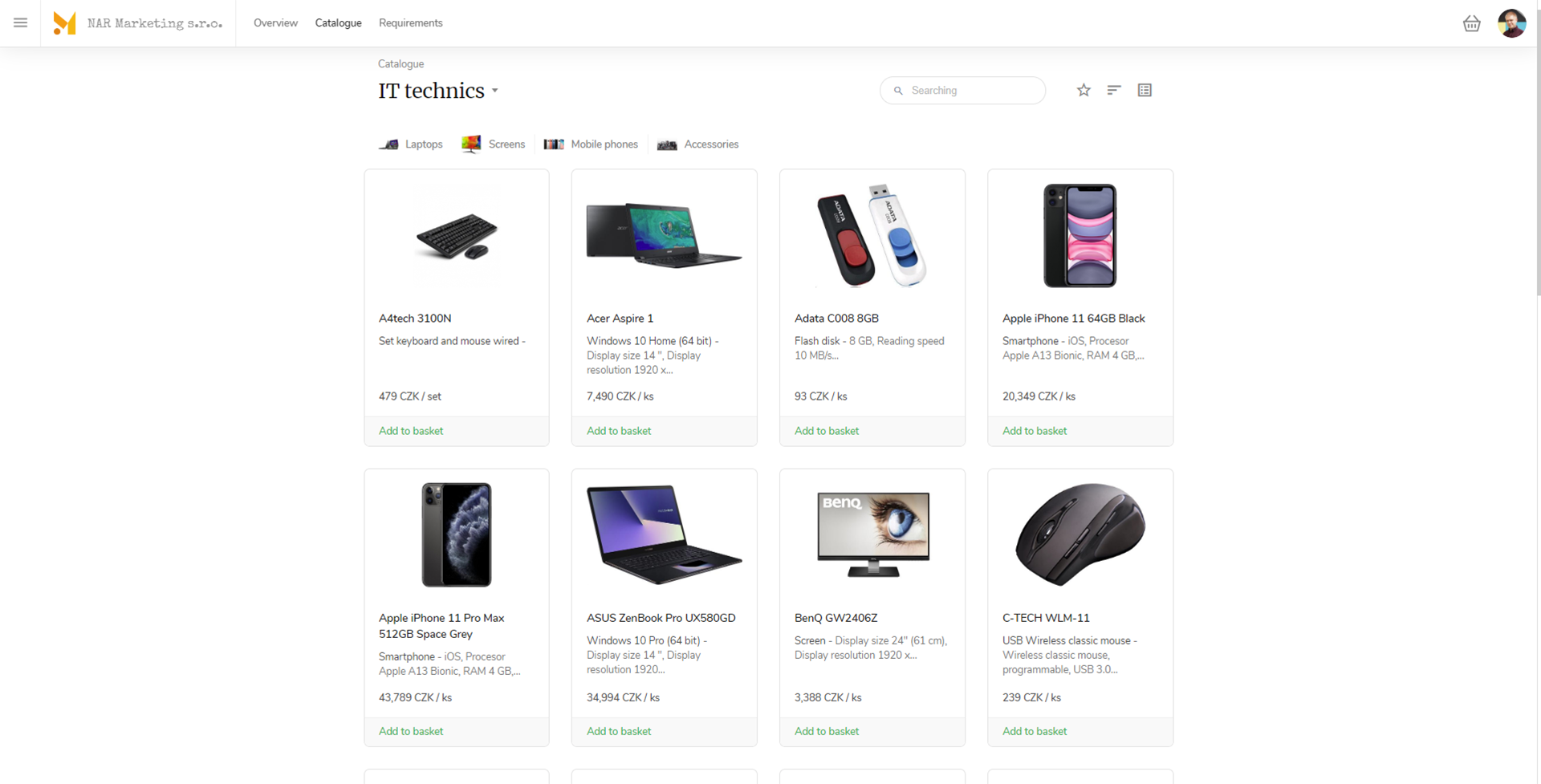A screenshot of a desktop website displaying a marketing page is shown. The interface features several tabs at the top, including "Overview," "Catalog," and an unreadable third tab, with the "Catalog" tab currently selected. The catalog displays various electronic devices arranged in rows of four items each. The first row includes an Acer Aspire laptop in the top right corner, a USB stick next to it, an Apple iPhone 11 on the far right, and a keyboard on the top left. The second row showcases an Apple iPhone 11 Pro Max, an Asus laptop, a BenQ monitor, and a Ctech mouse. The text on the screenshot is difficult to read, and the prices listed are in a foreign currency, not in dollars.